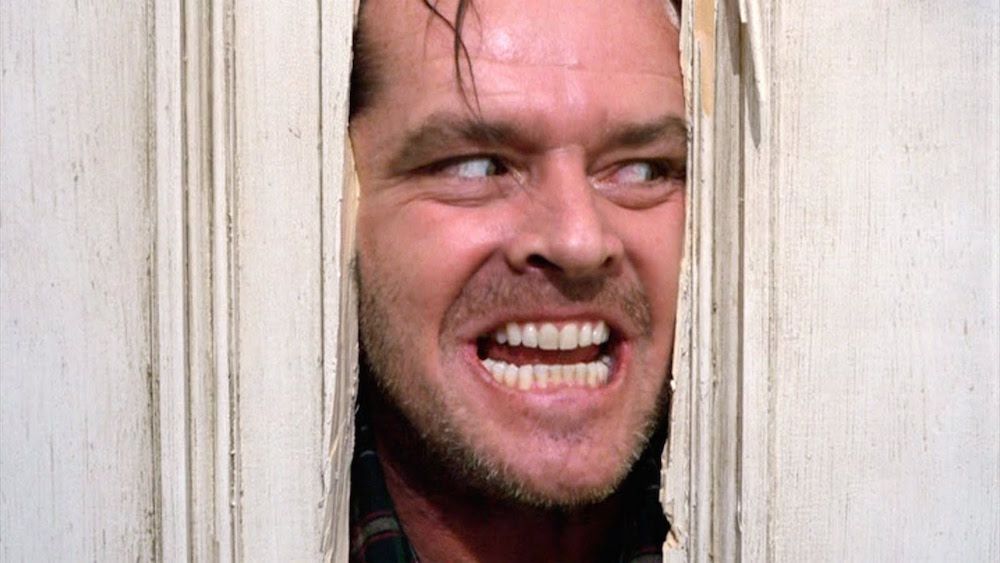This famous movie still from "The Shining" captures the iconic "Here's Johnny" scene featuring Jack Nicholson. The image shows Nicholson's face framed by broken, jagged pieces of a whitewashed door that he has just axed through. Nicholson is peeking through the narrow opening with a crazed expression, characterized by his reddish complexion, bushy eyebrows, and a few loose strands of hair falling over his forehead. He's baring all his teeth in a sinister grin, with his eyes wide and filled with madness, enhancing his terrifying look. He's wearing a green plaid shirt, visible through the door's gap. The intense scene depicts Nicholson's character about to break through the door completely, evoking a sense of imminent danger and urging any observer to run.